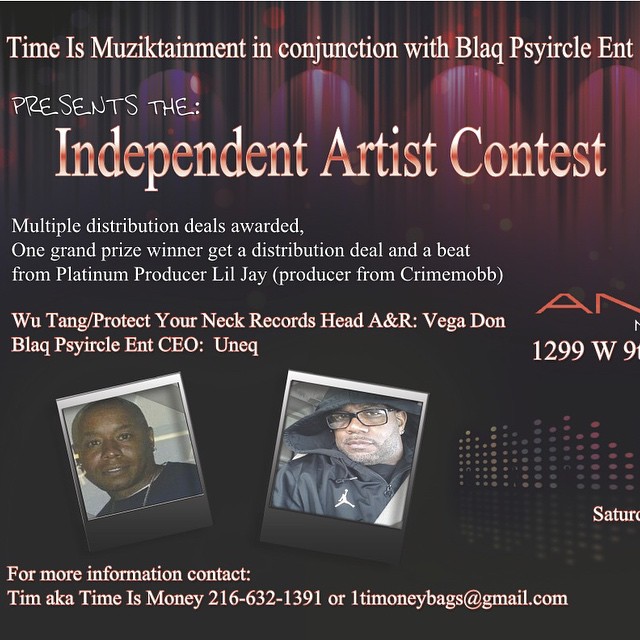This advertisement for the Independent Artist Contest features a digitally rendered curtain backdrop, reminiscent of an auditorium, with a vibrant color palette including black, brown, purple, orange, and white. The text overlay, in bold white font, announces the contest organized by "Time Is Music-Tainment" in collaboration with "Black Circle Ent." It highlights multiple distribution deals to be awarded, with one grand prize winner receiving a distribution deal and a beat from platinum producer Lil' J, known for working with Crime Mob. Additional collaborators include Wu-Tang/Protect Your Neck Records Head A&R Vigadon, and Black Circle Ent. CEO Eunik. At the bottom of the image, two Polaroid photos are centered – one of an African-American male in a dark blue shirt and the other of a Hispanic male wearing glasses and a black hoodie – likely representing key figures or producers involved in the contest. Contact information is provided for Tim, aka Timeismoney (216-632-1391 or onetimemoneybags@gmail.com) for further inquiries.